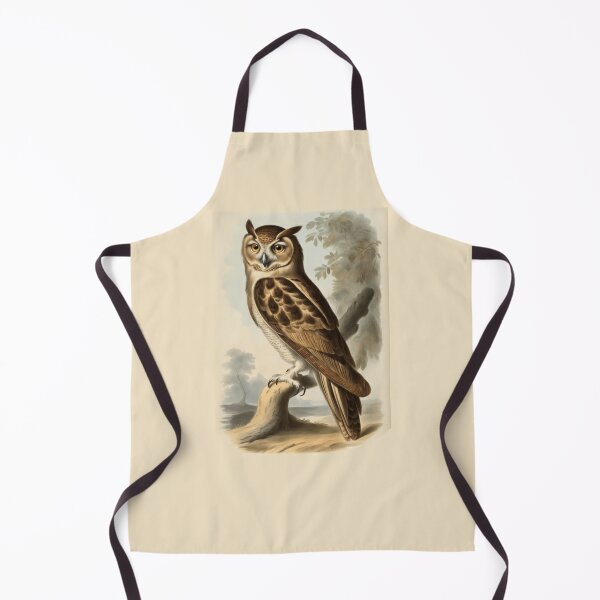This photograph features a light beige canvas apron meticulously placed on a plain white surface, giving it a sense of depth with subtle drop shadows. The apron is adorned with an intricately detailed illustration of a brown owl perched on a branch, in the style of an Audubon drawing. The owl is positioned to show its left side, though its face is turned toward the viewer, showcasing brown and tan feathers and a gray beak. The branch extends from the ground, surrounded by leaves and set against a backdrop of a blue sky. The apron’s neck strap, as well as its two long side straps, are a dark brown color and are laid across the apron in a relaxed S shape. The careful arrangement and striking owl illustration make this apron a standout piece, suitable for product imagery on a retail website.